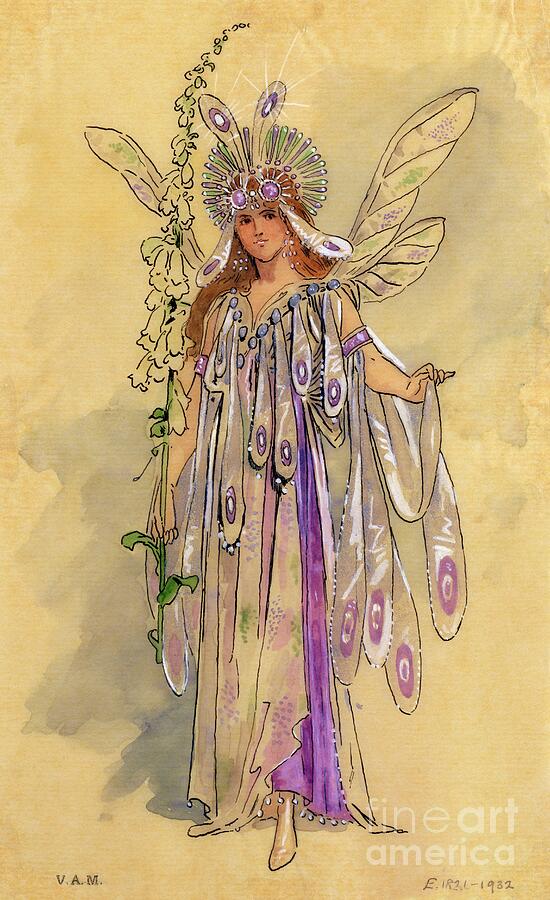The image depicts a fairy-like woman standing upright with long, flowing red hair. She is adorned with iridescent, transparent wings that display intricate patterns, featuring large peacock-like dots with smaller white circles at their centers. These wings, with hues of purple and green, are paired on each side, with one being longer and the other smaller. She wears an ornate headdress, also iridescent with purples and greens, and radiating rods that form a crown around her hair, along with additional petal-like elements that extend upwards and drape down by her cheeks, resembling feelers.

Her dress is a striking combination of various colors; primarily it is characterized by translucent fabric embellished with purple and green accents, similar to her wings. The garment features hanging elements that resemble ribbons or bands with purple spots, reminiscent of butterfly markings. The dress extends to her feet, revealing golden slippers at the bottom. She holds an ornate staff topped with numerous flowers matching her wings' color scheme.

At the base of the image, there is an inscription: "V.A.M" followed by letters and a date range "1821 to 1932." The overall visual effect is one of delicate, intricate beauty, capturing the ethereal essence of a fairy princess or goddess.